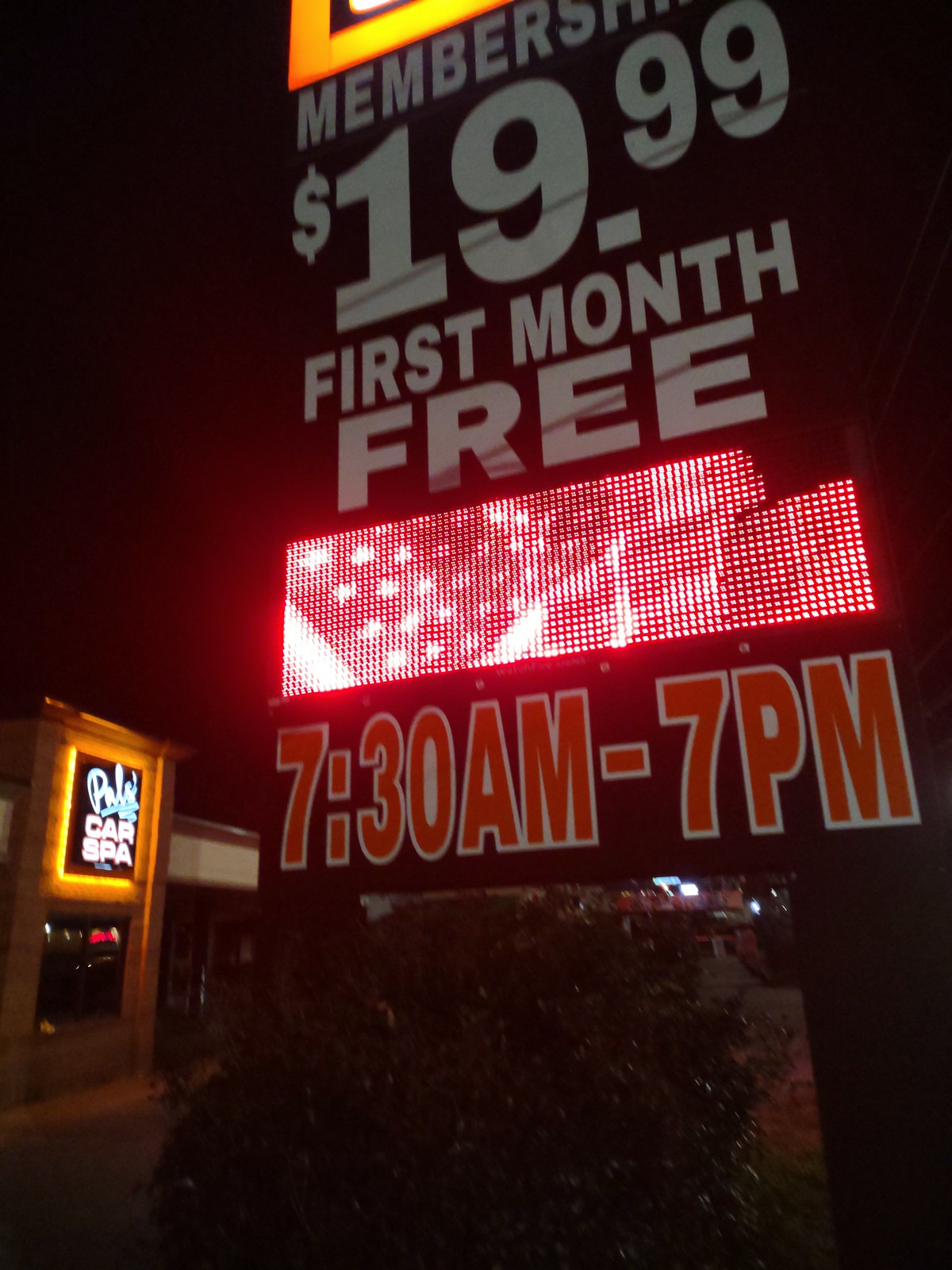This nighttime outdoor photograph captures a bustling scene dominated by a large illuminated sign and a nearby store. In the bottom left corner of the image, the store, identified as "Palo Car Spa," has a striking neon sign glowing with a yellowish-orange light. The words "Car Spa" are clearly visible and well-lit, positioned above a dark window. The surrounding area features a green bush, blending into the darkness. Towering above this setting, a large digital billboard takes center stage. The billboard displays a partially visible American flag image, accompanied by red pixelated lights. The top portion of the sign features a brightly lit section with white text stating, "Membership 1999 First Month Free." Below this, the operating hours "7.30am to 7pm" are highlighted in red letters. The top right corner of the billboard appears to be damaged, with some lights not functioning.